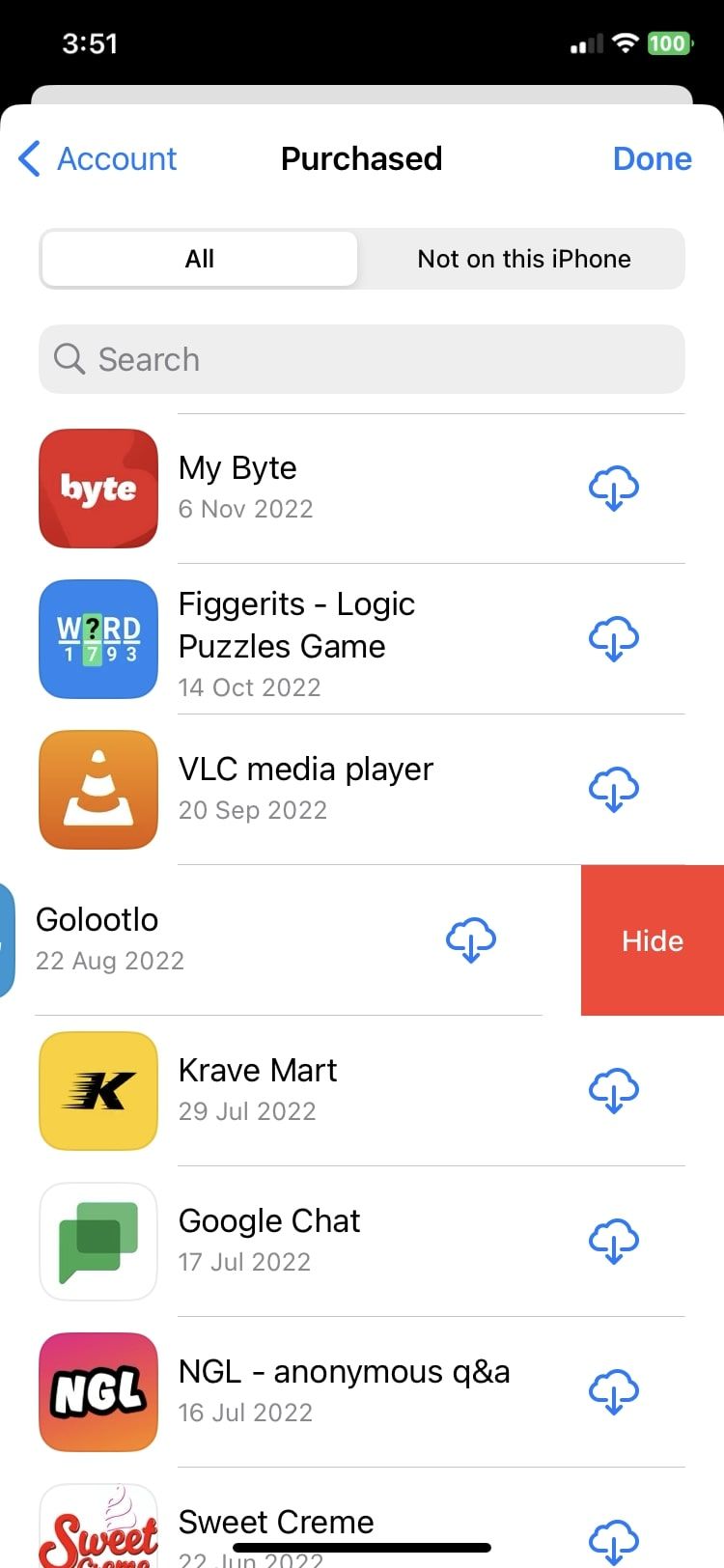This screenshot displays the interface of an iPhone's App Store under the 'Purchased' section. At the top right corner, the time is 3:51. The status bar indicates two bars of cellular coverage, active Wi-Fi, and a 100% battery level. The screen shows various tabs, with 'All' highlighted, alongside 'Account,' 'Purchased,' 'Done,' 'Not on this iPhone,' and a 'Search' option indicating the keyword 'my byte.' 

The first app listed is "Figgits" (logic puzzles game), downloaded on 14 October 2022, followed by "VLC Media Player" on 20 September 2022. The next entry is "Golootlo," listed on 22 August 2022. Adjacent to each app is a red rectangular button labeled 'Hide' in white text. Continuing down the list, "Crave Mart" is dated 29 July 2022, "Google Chat" from 17 July 2022, "NGL" (anonymous Q&A) on 16 July 2022, and "Sweet Creme" on 22 July 2022.

Each app entry also includes a blue cloud icon with a downward arrow on the far right, indicating that these apps can be redownloaded from iCloud. The image conforms to a portrait orientation, taller than it is wide, and there are no visible people in the screenshot.